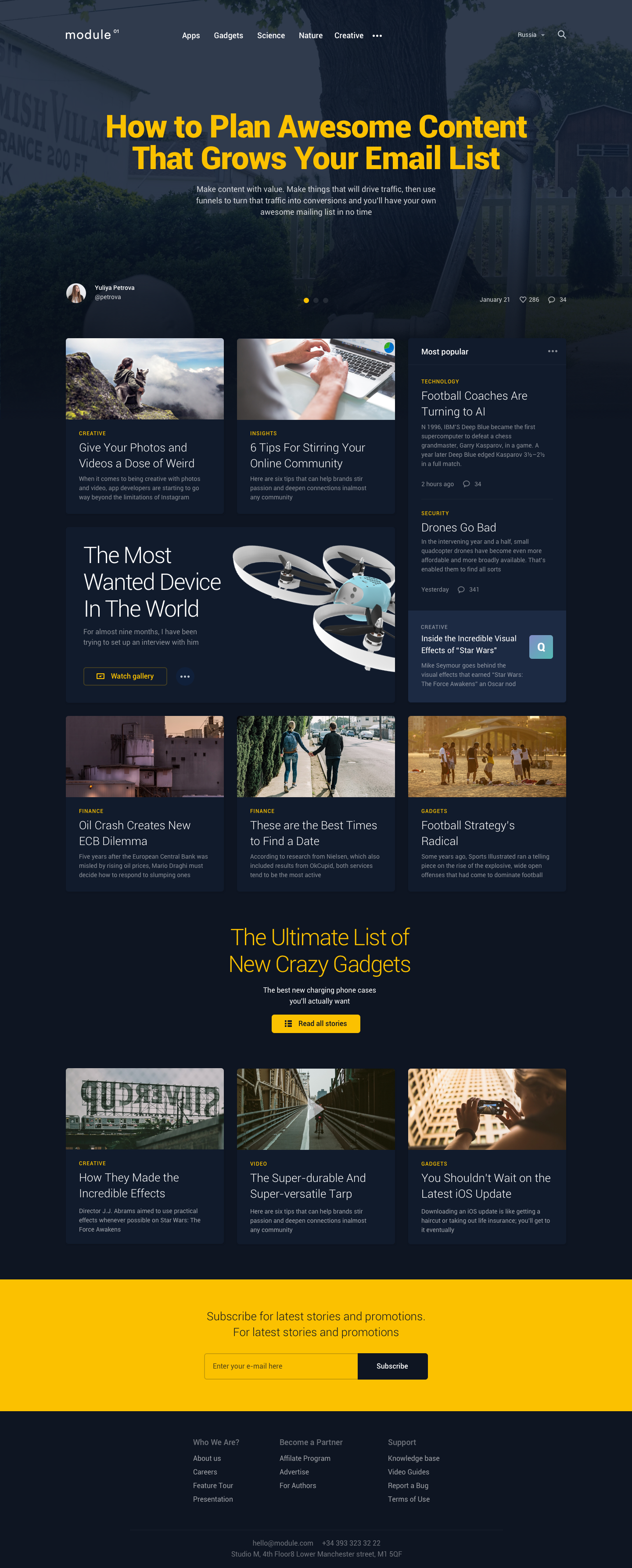The image has a vibrant blue background with the main title "How to Plan Awesome Content that Grows Your Email List" prominently displayed in eye-catching yellow text. Various pieces of information are presented in white text, organized around the image to capture viewers' attention effectively. 

In the upper left section, there's a profile picture of a woman placed alongside an inspiring scenic photograph of mountains, paired with relevant descriptions. Below this, there is a photograph of a person typing on a keyboard, suggesting productivity, with adjacent text details.

Towards the center-right, there's an enticing headline about "The Most Wanted Device in the World," accompanied by an image of a stylish home interior, adorned with informative content. Adjacent to this, an engaging photo depicts two men standing at the edge of a cliff with more descriptive text.

Further down, smaller groups of people are seen near what appears to be an outdoor shelter, and this section contains additional information organized around the visual elements. Highlighted prominently in yellow is the eye-catching title "The Ultimate List of New Crazy Gadgets."

At the bottom, the layout features three square photos next to informational text, forming an intuitive and engaging grid. A striking yellow rectangle featuring a box graphic is adjacent to a blue rectangle with the word "Subscribe" in bold white letters, encouraging user engagement effectively.